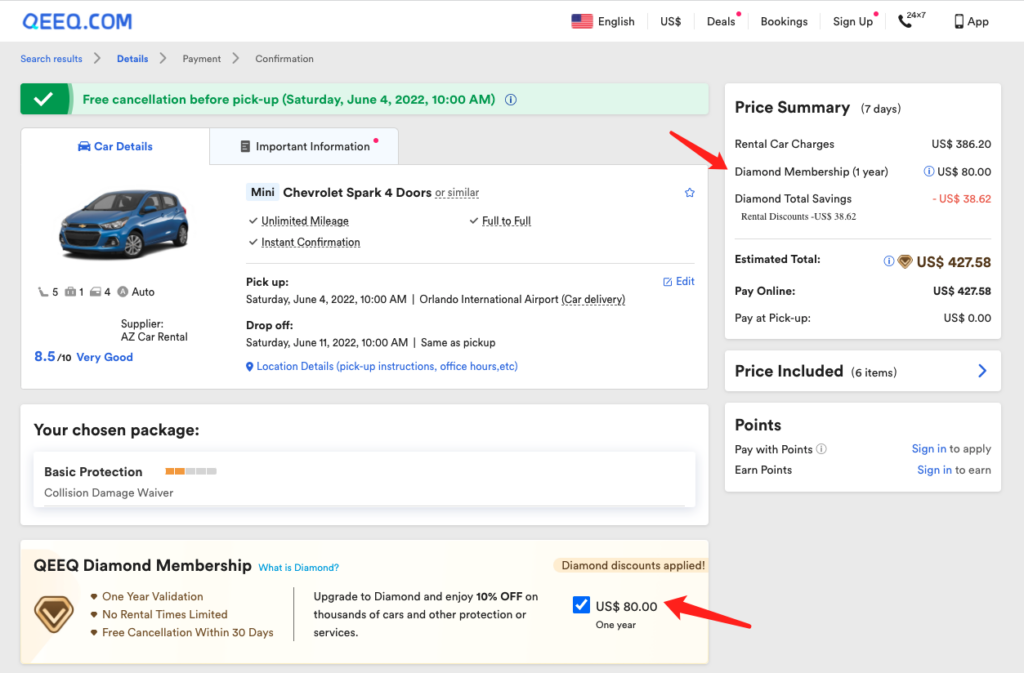The screenshot features the QEEQ.com website, showcasing a rental car booking interface.

At the top, there's the QEEQ logo in royal blue text, accompanied by a series of icons and options aligned horizontally:
1. An American flag followed by the text "English" and a vertical light gray line.
2. "US dollars" preceded by another vertical gray line.
3. "Deals" with a small red dot above the 'S', again separated by a vertical gray line.
4. "Bookings" followed by a gray line.
5. "Sign up" with a red dot above the 'P' and another vertical gray line.
6. "24 by 7" accompanied by a phone icon, indicating round-the-clock support.
7. An icon labeled "App".

The background is predominantly white, transitioning into a gray section where the menu path is displayed: "Search Results > Details" in blue, hinting at active navigation, followed by grayed-out "Payment" and "Confirmation".

Within the gray box, a green box with a white checkmark states "Free cancellation before pickup Saturday, June 4th, 2022, 10 a.m.", including an information button. Below this is a detailed description of the booking:
- Vehicle: Mini Chevy Spark or similar, a four-door vehicle, unlimited mileage, instant confirmation, full-to-full fuel policy.
- Specifications: Seats five passengers, accommodates one piece of luggage, automatic transmission, rated 8.5 out of 10 (Very Good).
- Pickup Details: Scheduled for Saturday, June 4th, 2022, at 10 a.m. from Orlando International Airport.
- Dropoff Details: Scheduled for Saturday, June 11th, 2022, at 10 a.m., same location.
- Additional Information: Location details, pickup instructions, office hours provided via an editable link icon.

A highlighted membership section explains QEEQ Diamond Membership:
- Benefits include one year of validation, no rental time limitations, and free cancellation within 30 days.
- Upgrade option offers a 10% discount on thousands of cars and additional services, costing $80 for the year.
- An active diamond membership application is displayed, with marked-up red arrows pointing to the membership details in the price summary.

The price summary includes:
- 7-day rental car charges: $386.20
- Diamond membership fee for one year: $80
- Total savings from the diamond membership: $38.62
- Estimated total cost: $427.58, to be paid online, with zero payment at pickup.

A final box presents options for points:
- "Pay with points" and "Sign in to apply or earn points".